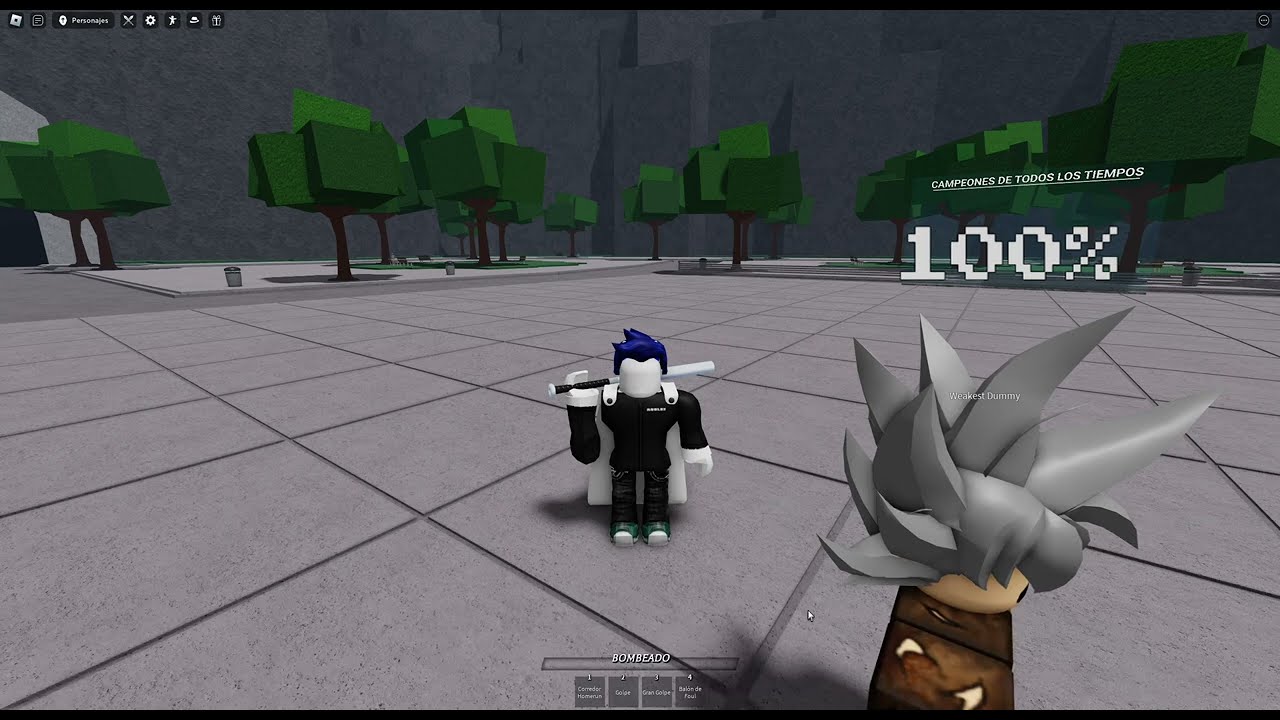This is an image from a Minecraft-style video game depicting a courtyard-like area with large, gray, square tiles as the ground. In the background, a tall, dark gray wall stands behind a row of green, blocky trees with brown trunks. The scene features two characters in the foreground. The central character, resembling a Lego figure, has white skin, short blue hair, and a white face with low-set features. This character wears a black outfit with patterned black pants and green shoes, and carries a black and white stick on their shoulder. The second character, seen partially and from the side, has a cream-colored complexion with spiky gray hair, wearing tattered brown clothing. At the bottom middle of the screen, text reads "Bombiato," accompanied by the numbers 1, 2, 3, and 4, indicating some form of stats. Above the second character, white text in Spanish reads "Campeones de Todos los Tiempos 100%," and in the lower right-hand corner, additional text states "Weakest Dummy."